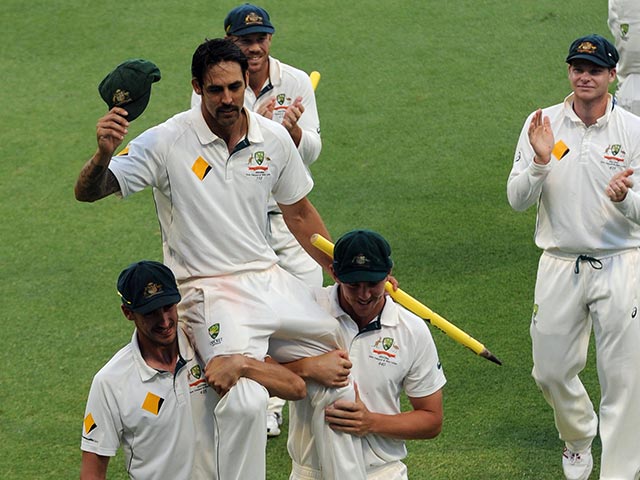In the image, five men are seen celebrating a victory on a green field, likely a cricket match judging by their uniforms and paraphernalia. They are all dressed in white uniforms, consisting of white sweatpants and either short-sleeve or long-sleeve polo tops branded with a green crest featuring a kangaroo and an emu, suggesting they are from Australia. The front of the scene captures two men who are carrying a third man on their shoulders. The raised man, sporting a mustache, has removed his green cricket cap and is waving it in his right hand while holding a yellow spike, probably a wicket, in his left hand. Meanwhile, the two men carrying him, who also wear green caps, are joyfully looking down towards the camera. Behind them, another man, also with a mustache and wearing a green cap, is clapping and smiling. To his left stands a man in a long sleeve shirt, with his hands apart as if he just finished applauding, and his right knee slightly bent. The jubilant expressions and celebratory posture of all five men indicate they are commemorating a significant victory, further supported by their matching white uniforms and green caps.